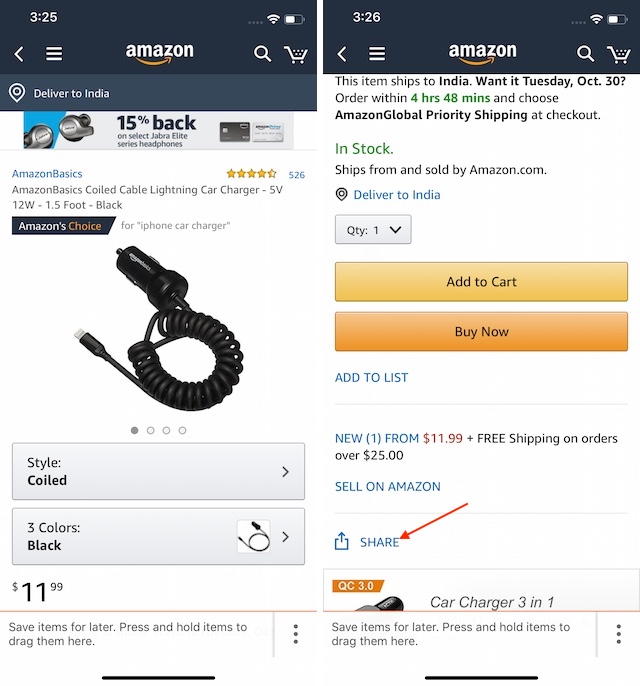The image comprises two screenshots taken from a cell phone displaying the Amazon Prime app. At the top of the screen, a black banner features the Amazon Prime logo with "Amazon" in white and the signature orange smile. The first screenshot displays an advertisement for Amazon Basics Cold Cable Lightning Car Charger. This ad highlights a 15% cashback offer and includes images of relevant credit cards.

The promoted item is the "Amazon Basics Cold Cable Lightning Car Charger" with specifications of 5 volts, 12 watts, and a 1.5-foot length, available in black. The image shows one of four selectable pictures, with the first one currently highlighted. Additional options at the bottom of the screen include style selections and three color choices. The price is listed as $11.99.

The second screenshot appears to be a continuation of the product page, showing more detailed information as if the user has scrolled down. It confirms availability with "In Stock" status and provides purchase options such as "Add to Cart," "Buy Now," and "Add to List." It notes that the item is new and offers free shipping on orders over $25. A red arrow has been drawn to emphasize the "Share" option, suggesting instructional guidance on how to share the item on Amazon.